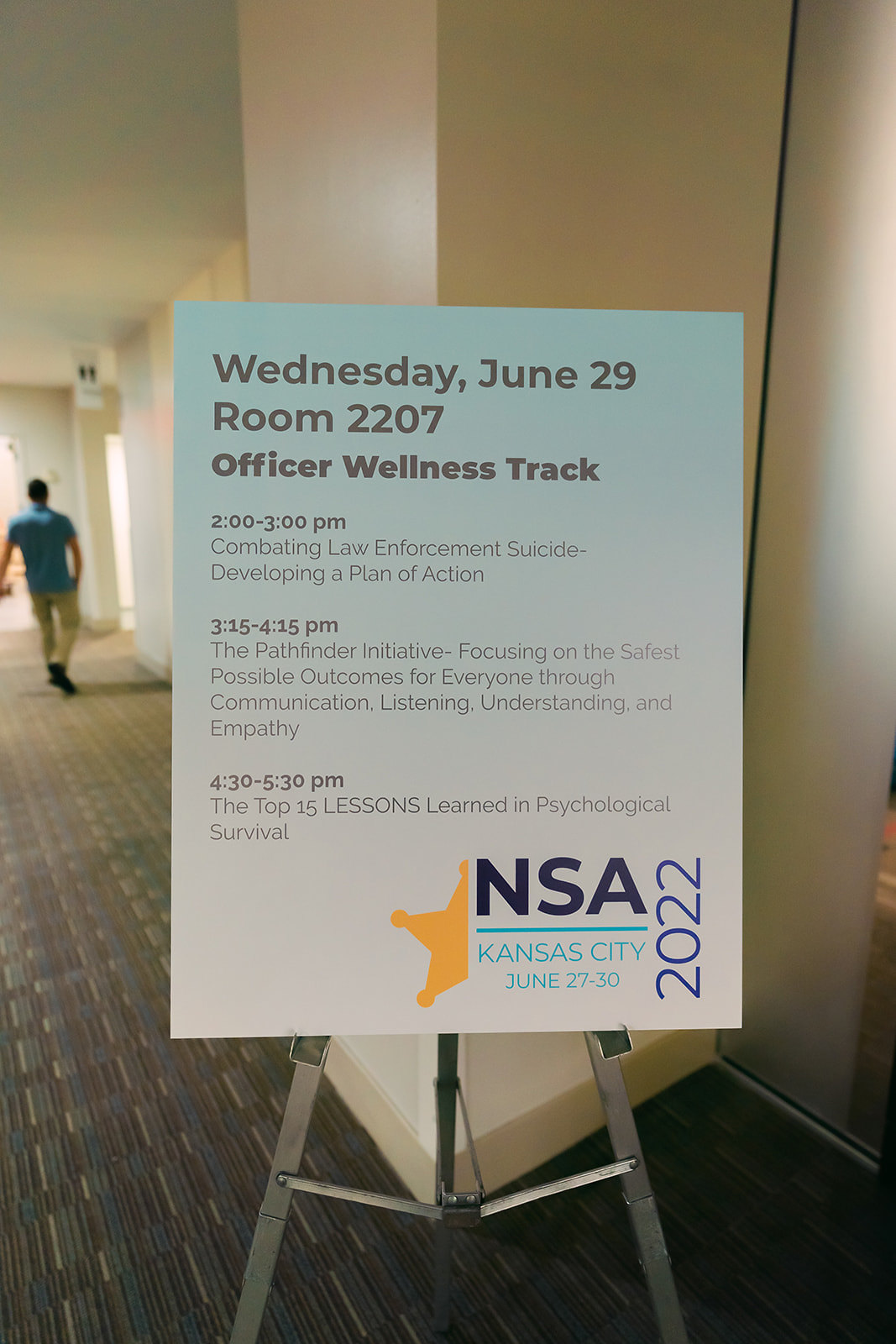This is a detailed photo of a white paper or cardboard sign displayed on a tripod in a carpeted hallway, likely within a hotel conference center. In the background, there is a person wearing a blue shirt and tan pants, walking away and appearing blurry. The sign, headed "Wednesday, June 29, Room 2207," lists events for the Officer Wellness Track: 

- From 2 to 3 p.m., "Combating Law Enforcement Suicide: Developing a Plan of Action."
- From 3:15 to 4:15 p.m., "The Pathfinder Initiative: Focusing on the Safest Possible Outcomes for Everyone Through Communication, Listening, Understanding, and Empathy."
- And from 4:30 to 5:30 p.m., "The Top 15 Lessons Learned in Psychological Survival."

At the bottom of the sign, it notes "NSA, Kansas City, June 27 to 30, 2022," accompanied by an image of half a star, designed to resemble a sheriff's badge with rounded points.